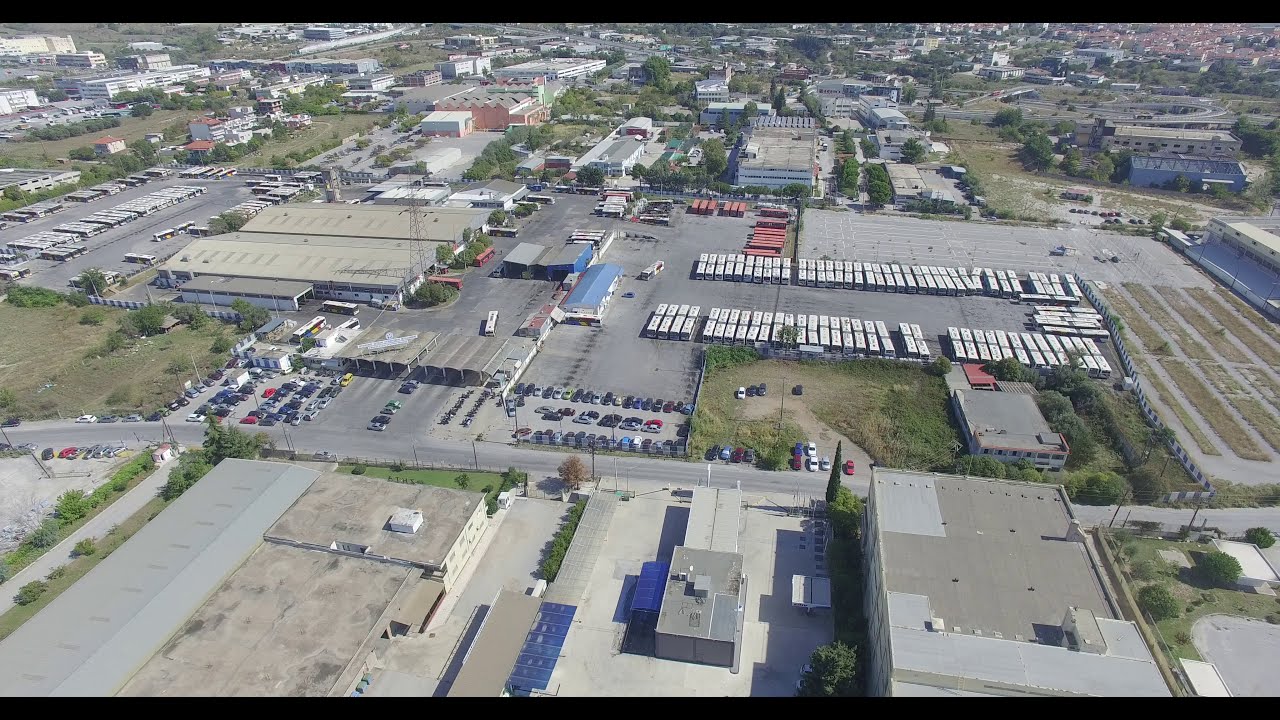The aerial image captures an expansive industrial area within a city, interspersed with a variety of buildings and greenery. Centrally positioned at the bottom are several industrial buildings characterized by grayish tan, white, and salmon-colored exteriors. In the middle of the image lies a sizable parking lot populated with cars in a spectrum of colors—red, yellow, blue—along with several buses featuring white tops and some trailers with red tops. Surrounding the parking lot and spreading into the background, the industrial landscape transforms into an array of structures, including low one-story white buildings with dark rooftops and a few multi-story gray-roofed buildings interspersed with red brick structures. Green fields, trees, bushes, and other patches of vegetation permeate the scene, adding a natural contrast to the urban sprawl. The backdrop extends further into the cityscape, dotted with more buildings. Notably, there's an area that could be a school or similar institution, identified by clusters of buses or trailers. No text disrupts the view, and the aerial perspective offers a comprehensive, detailed overview of this multifaceted industrial park.